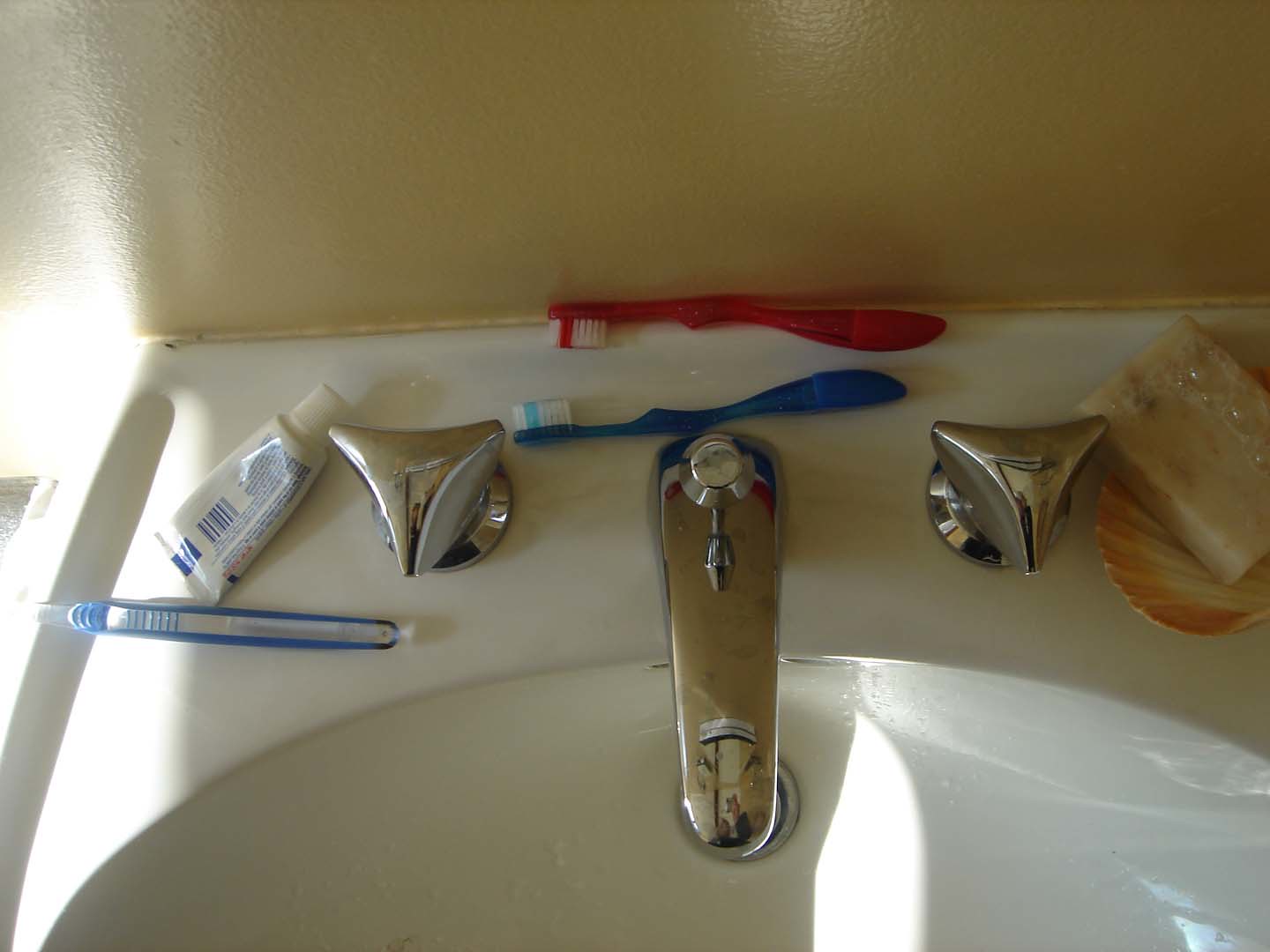The image showcases the top part of a white porcelain bathroom sink, focusing on its faucet and knobs. The faucet, which has a somewhat old appearance, is flanked by two ergonomically triangular knobs—one for hot water and the other for cold. Resting on the sink's surface, adjacent to the faucet, is a small sample-sized toothpaste tube, white with blue text and barcodes, positioned upside down. There are three toothbrushes: one clear with blue trim, another red, and a blue one identified as likely from Oral-B. The red toothbrush leans against a tan wall, while the blue toothbrush sits in front of it. On the right side of the faucet, a soap dish shaped like a clam shell holds a bar of soap with visible bubbles. The image captures the upper section of the sink, emphasizing the arrangement of dental and hygiene items around the faucet area.